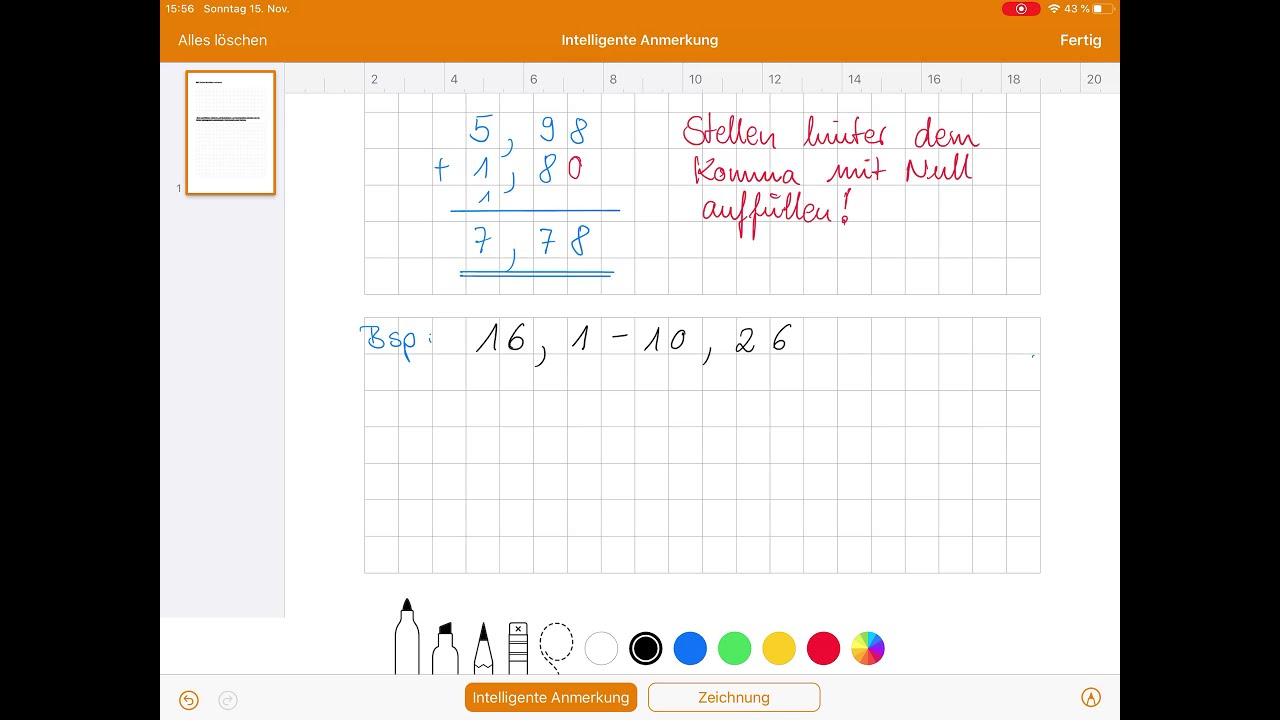The image depicts the screen of a digital note-taking application, likely on an iPad or iPhone, showcasing a white background of graph paper. The screen features a grid pattern composed of little gray squares and is sectioned into four areas designated for graphs. At the top of the screen, there is an algebra equation followed by its solution beneath it. Adjacent to the equation on the right, in red cursive, are notes written in German. The header of the screen reads "Intelligente ANMERKUNG," and the upper-right corner displays "FERTIG," with icons indicating WiFi connectivity and battery level beside it.

The main image area displays mathematical formulations alongside German text, including phrases such as "STELLEN BIUTER DEM," "KAMUA MIT null," and "AUFFUILLEN!" Subsequent to these phrases are combinations of letters, numbers, and symbols like "5 G8 V 8 0," "7 7 8," "BSP V 6 V- V 0, 26." At the bottom of the screen, there is a toolbar providing various marker tool options, allowing users to adjust the width and color, with choices including black, blue, green, yellow, red, and a multi-color option. Additionally, it displays tools resembling a marker, pencil, and highlighter.